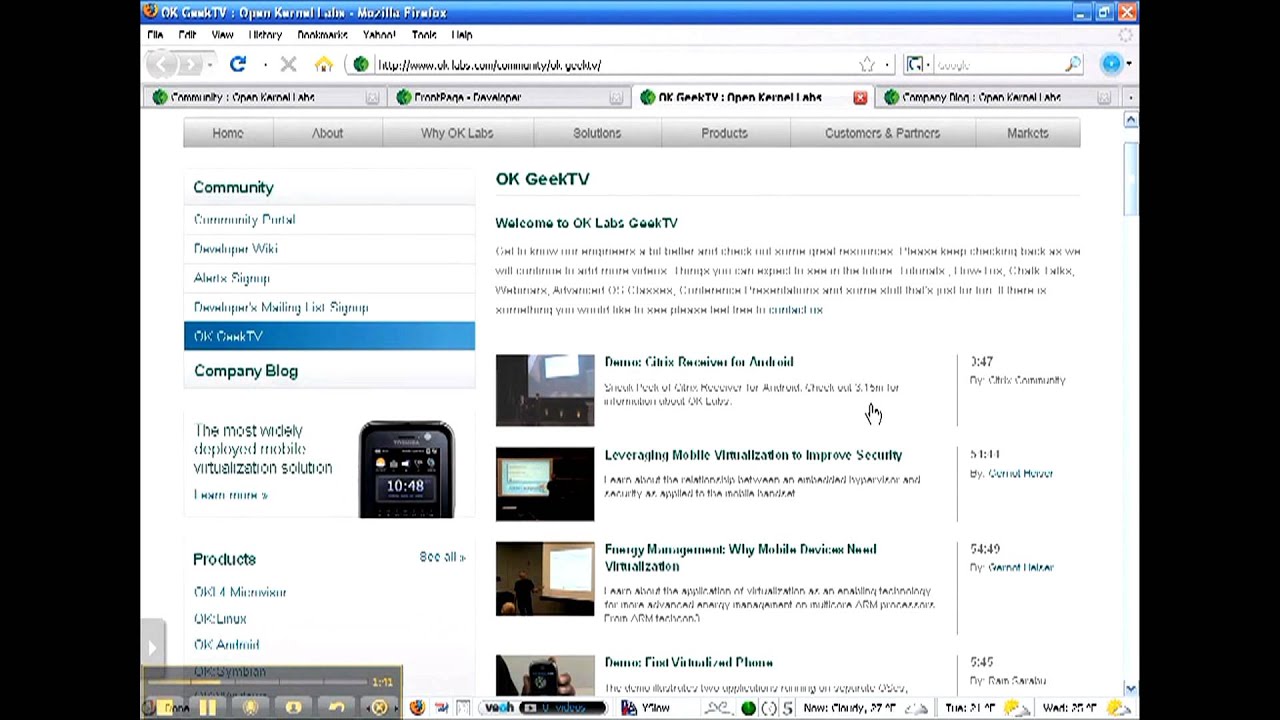Screenshot of a Firefox web browser displaying the homepage of the website "OK Geek TV." The browser interface shows the standard menu options (File, Edit, View, History, etc.) at the top, followed by the URL bar and tab section. The main content area features the "OK Geek TV" Homepage with a heading that reads "Welcome to OK Labs Geek TV," though the latter part of the heading is hard to decipher. The page appears to contain a series of tutorials or video thumbnails, with a sidebar on the left that includes a "Community" tab and various posts. The website likely serves as a platform for sharing information and tutorials, possibly geared towards individuals who repair monitors, TVs, and similar electronic devices.